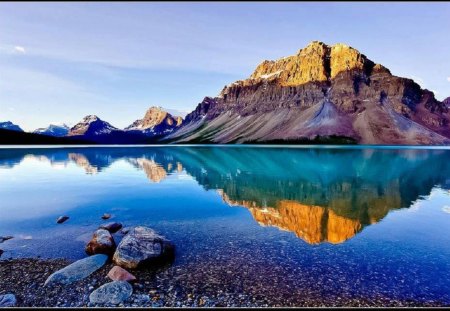The image captures a tranquil, picturesque mountain range reflected in a serene, brilliantly blue lake. Dominating the right side of the photo is a large mountain, its brown and snow-capped peaks basking in a mix of sunlight and shadow. To the left, two smaller mountains, along with an even smaller one further left, form a harmonious backdrop, all mirrored impeccably in the lake's glassy surface. The lake's water near the shore reveals a light blue-green hue, transitioning to a darker blue further out. The foreground displays a gravelly shore interspersed with dark brown rocks, adding texture and depth. The richly detailed reflection shows the mountains' varying hues—from yellow sunlight kissed peaks, through shadowed brown rocks, to sunlit sands. These elements are set under a light blue sky with sparse, wispy clouds, enhancing the natural, calming effect of the scene.